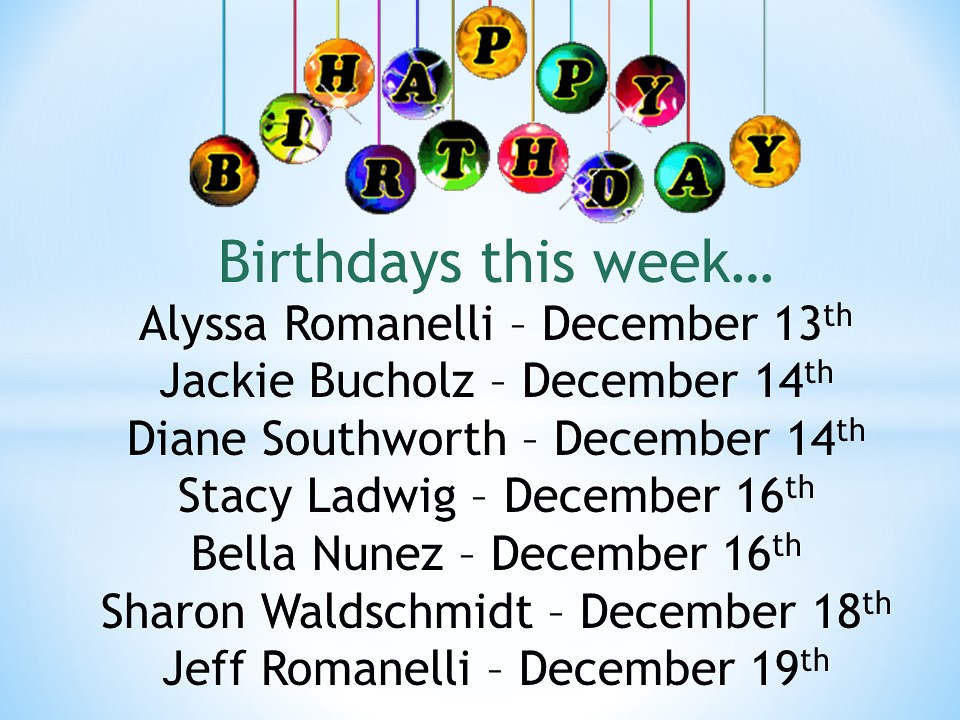The image is a rectangular banner with a light blue background, accented with transparent white patches to simulate clouds. The center of the image transitions to a bright white, mimicking the brightness of the sun. 

At the top of the banner, multicolored ornament-like balls hang from strings, each letter of "Happy Birthday" displayed within a ball. The letters are in black print with gold outlines: the 'H' is in a gold ball, 'A' in a purple ball, the first 'P' in a gold ball, second 'P' in a green ball, third 'P' in a red ball, 'B' in a goldish ball, 'I' in a combination of green and purple balls, 'R' in a purple and blue ball, 'T' encircled in green and white, with additional pink and purple balls adorned with star-like glints. The 'A' is housed in a green ball, and 'Y' in a gold or yellow ball.

Below this decorative text, the phrase "birthdays this week..." is centered and written in bluish-green print. Further down, a list of names and dates in black print on a white background features:

- Alyssa Romanelli - December 13th
- Jackie Buchholz - December 14th
- Diane Southworth - December 14th
- Stacey Ladwig - December 16th
- Bella Nunez - December 16th
- Sharon Waldschmidt - December 18th
- Jeff Romanelli - December 19th